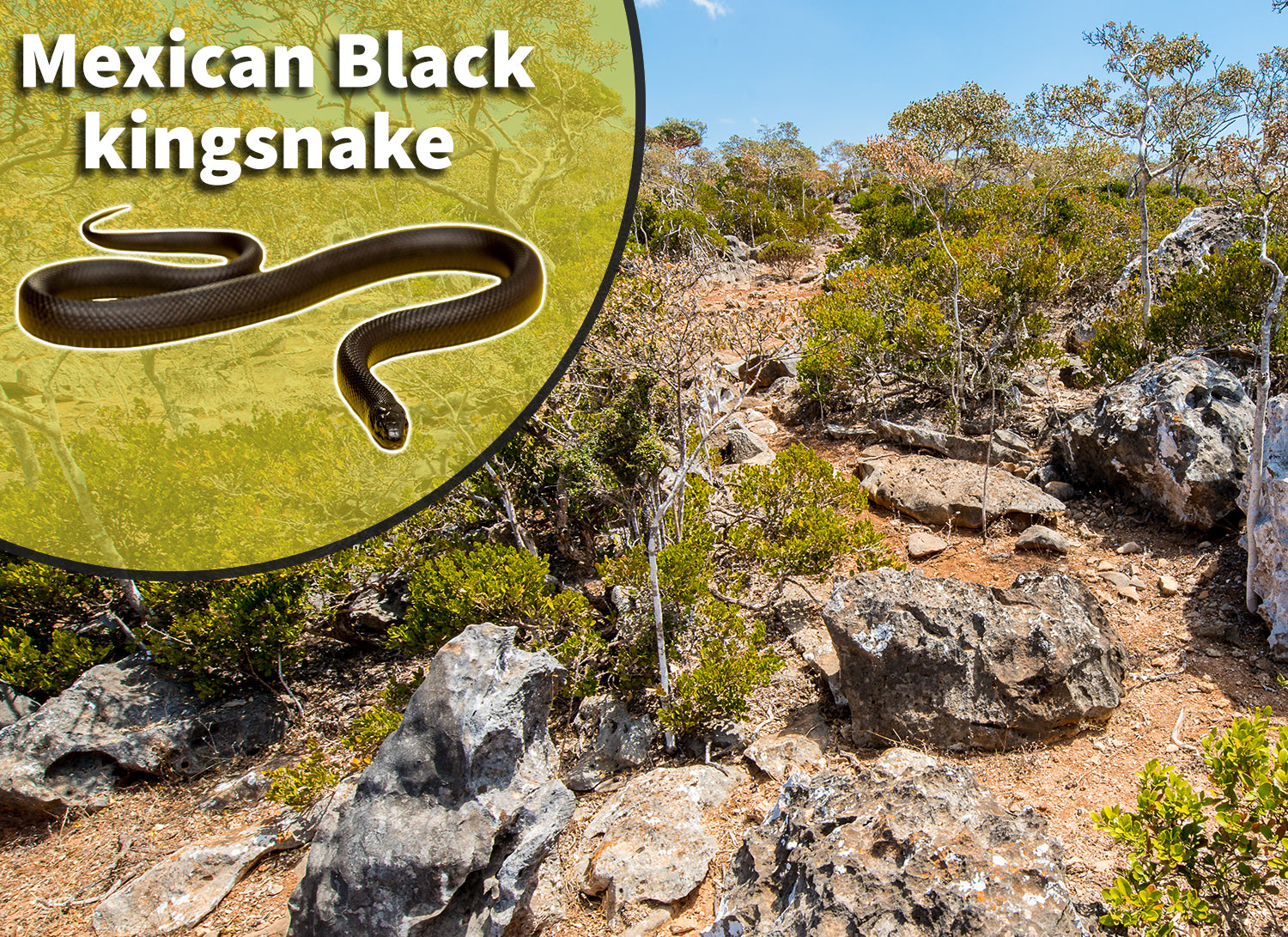This photograph captures a semi-arid landscape, characterized by an array of large, jagged boulders in shades of gray and tan, small trees, and sparse bushes. Amidst this desert-mountain hybrid region, a Mexican Black Kingsnake is presumably present, though it remains well-camouflaged and difficult to spot against the rocky terrain. Highlighting its elusive nature, there is a partially visible yellowish-green semicircle with a black outline in the top left corner. This semicircle contains white text reading "Mexican Black Kingsnake," with "Mexican" and "Black" capitalized and split across two lines, featuring a drop shadow for emphasis. Also within the semicircle is an illustrated black snake facing toward the viewer. Despite the snake's dark color, it blends seamlessly into the photograph's backdrop, adding to the intrigue and challenge of identifying its exact location among the rocks and vegetation.